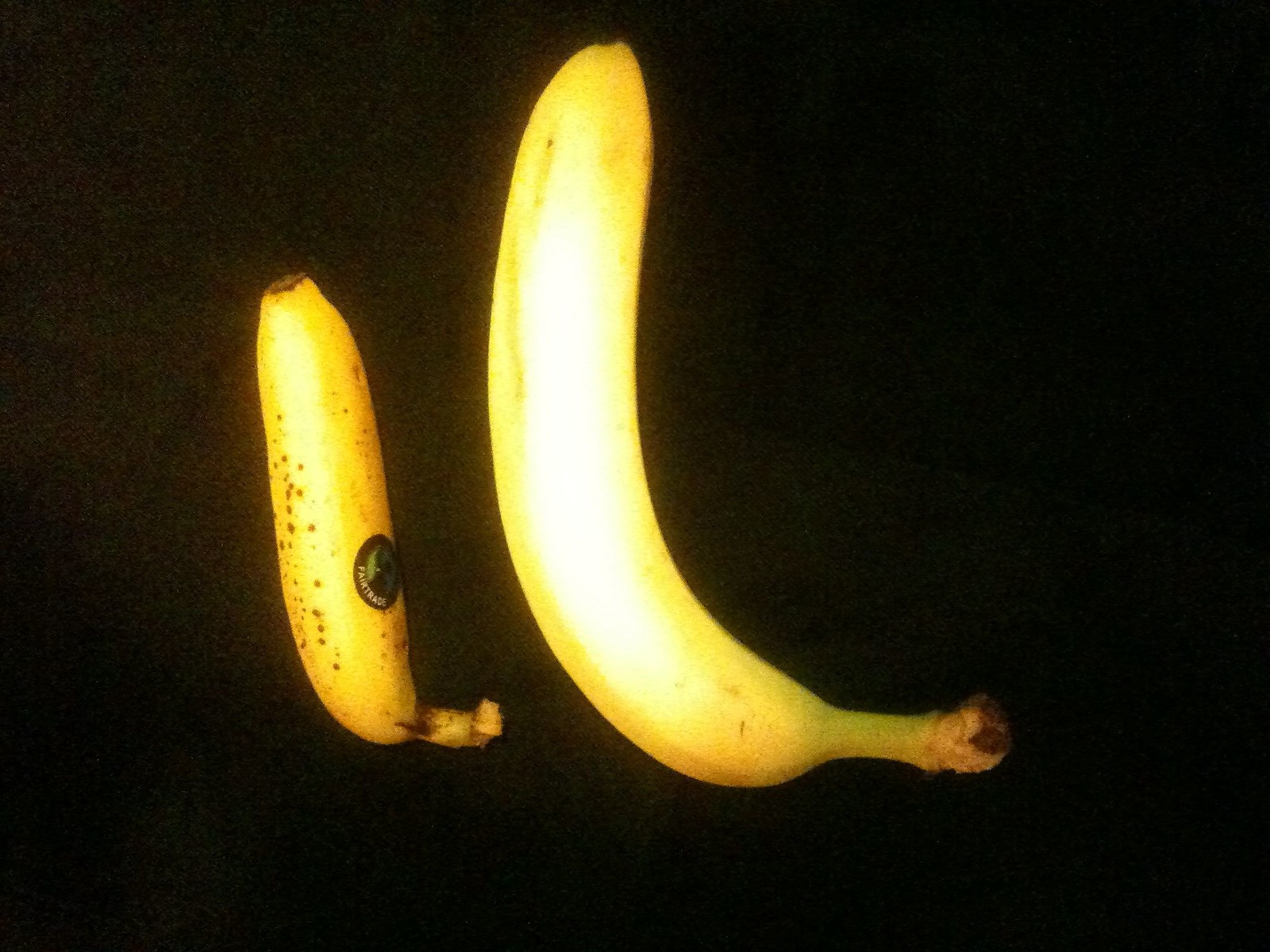The image showcases two bananas positioned upright with their stem ends on the bottom, lying horizontally to the right. The banana on the right is significantly larger and taller than the one on the left, which is adorned with a sticker on its lower half. The smaller banana on the left has a few brown spots and a shorter stem compared to the elongated stem of the curvier, larger banana. The taller banana's pronounced curve catches sunlight, creating a white glare on its surface. The backdrop of the image is a deep black, contrasting with the bright yellow of the bananas.